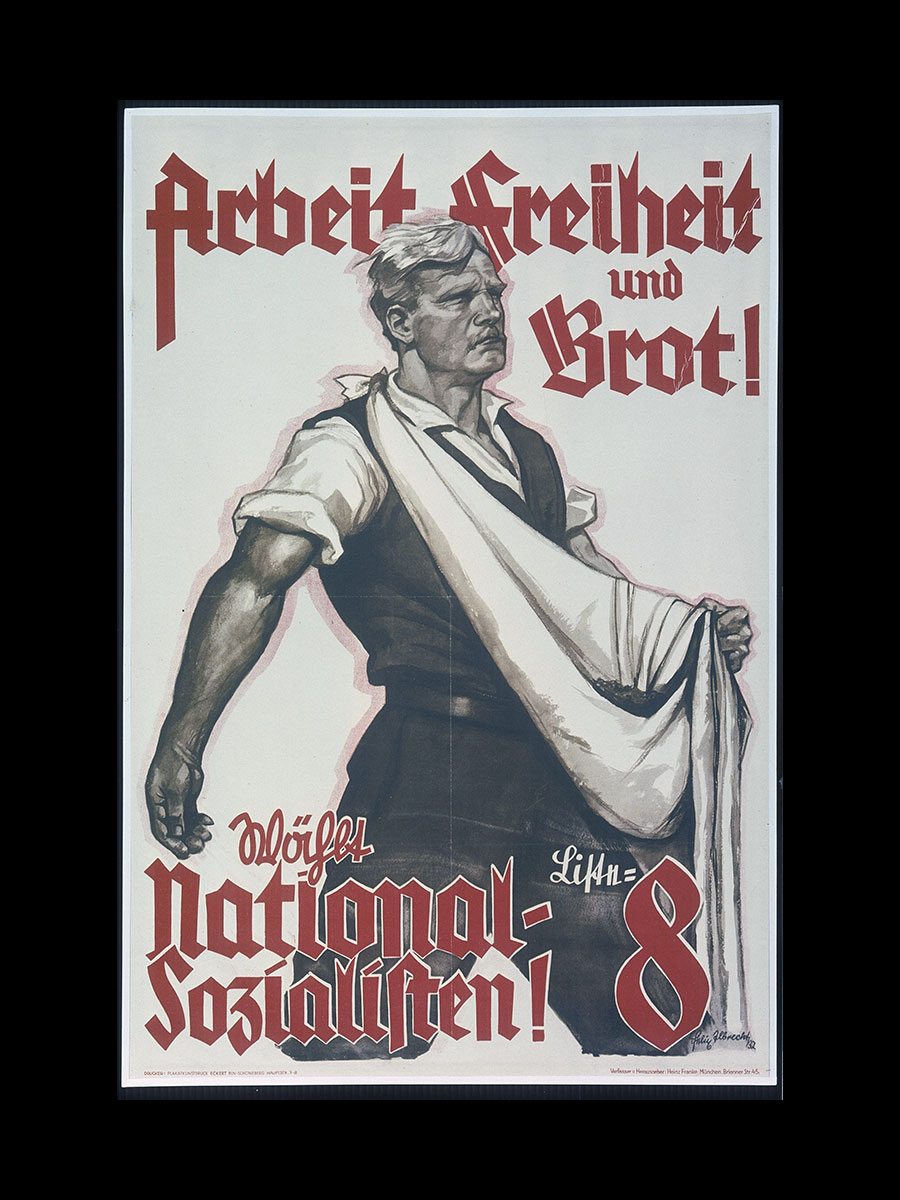The image is of an illustrated German poster, likely the cover of a magazine or comic book. The design features a middle-aged man with a mustache and flowy hair, wearing a white collared shirt with sleeves rolled up to his biceps, a black vest, black pants, and a black belt. The man appears muscular and is depicted with a stoic expression, gazing into the distance. His left arm is in a white sling, which is wrapped around his neck. The illustration is rendered in graphite, using a simple color palette of black, white, and red. The red German text, styled in gothic script, is prominently displayed above and below the image, with a red number 8 indicating the issue number at the bottom right corner. The overall composition is eye-catching and minimalist, set against a black frame.